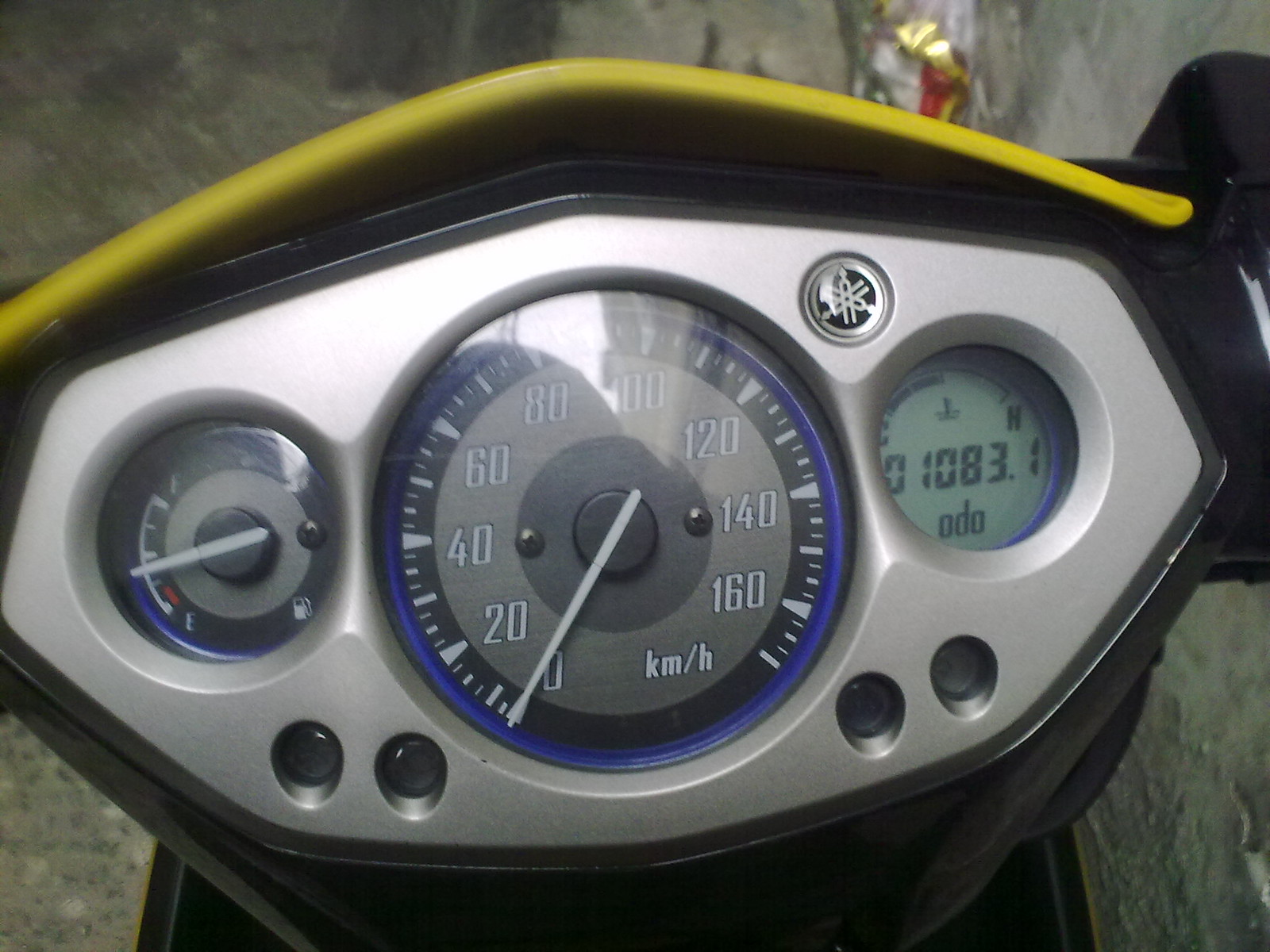The photograph showcases the front console panel of a scooter, characterized by its silver background and an oval-shaped design with a black base. Dominating the center of the panel is a large, circular speedometer, displaying white numbers encircled first by a black ring and then a blue ring. The speedometer, calibrated in kilometers per hour, currently points to zero. To the left of the speedometer lies the fuel gauge, detailing a quarter tank of gas, close to the red empty zone. This gauge also features a small fuel pump illustration.

On the right side of the panel resides a digital odometer, indicating a reading of 01083.1. Just above the odometer, the company logo is visible, as well as a portion of the scooter's yellow paint. Below these central elements are the turn signal indicators, which are currently off. The entire setup is mounted against a backdrop that includes a hint of cement, further emphasizing the scooter's outdoor environment.